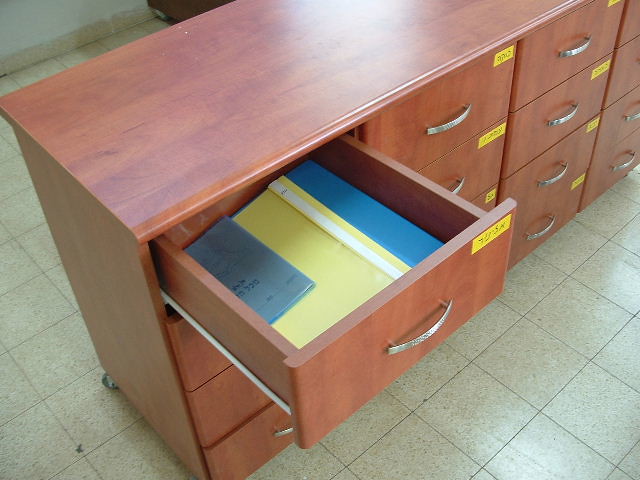The image showcases a medium-colored wooden cabinet with a polished finish, resting on a tiled floor featuring pale, gray, and black speckles with a cream background. The cabinet, which has several drawers arranged in columns, is equipped with sleek, silvery metal handles and is mounted on wheels. The topmost drawer on the left side is open, revealing its contents: a light blue book, blue and yellow file folders, and some papers. Each drawer in the cabinet is labeled in the upper right corner with a piece of yellow tape containing text. The cabinet drawers operate on roller-assisted slide-outs, visible from the open drawer's railing mechanism. The background of the image includes a partial view of a white wall in the upper left corner.